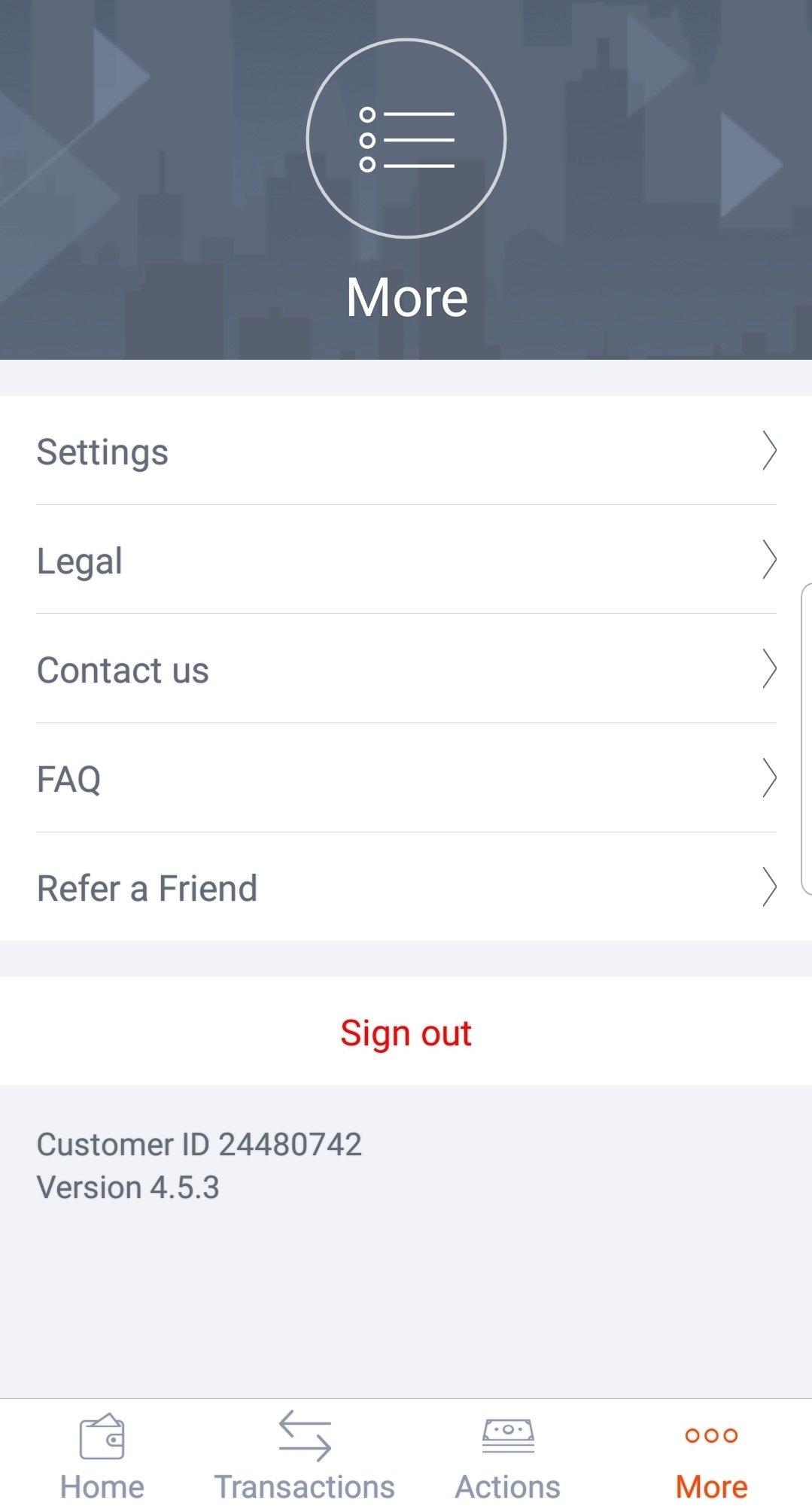This image is a detailed screenshot from an unidentified digital interface. The top portion features a gray rectangle adorned with an abstract design. Central to this rectangle is a thin white circle enclosing a bullet point list, accompanied by the text “More” beneath it.

The main body of the screenshot consists of a white background displaying various menu options: 

- “Settings”
- “Legal”
- “Contact Us”
- “FAQ”
- “Refer a Friend”
- “Sign Out”

Additionally, there is identifying information including:
- “Customer ID 24480742”
- “Version 4.5.3.”

The lower segment of the interface contains navigation icons paired with text labels:
- An icon resembling a wallet with the label “Home.”
- An icon depicting arrows pointing left and right labeled “Transactions.”
- An icon of a dollar bill with the label “Actions.”
- Three open red circles above the word “More.”

The entire image is vertically oriented, lacks any photographic elements, and does not include people, animals, birds, plants, vehicles, or any other objects. It purely consists of graphical and text elements typical of an app or web interface.